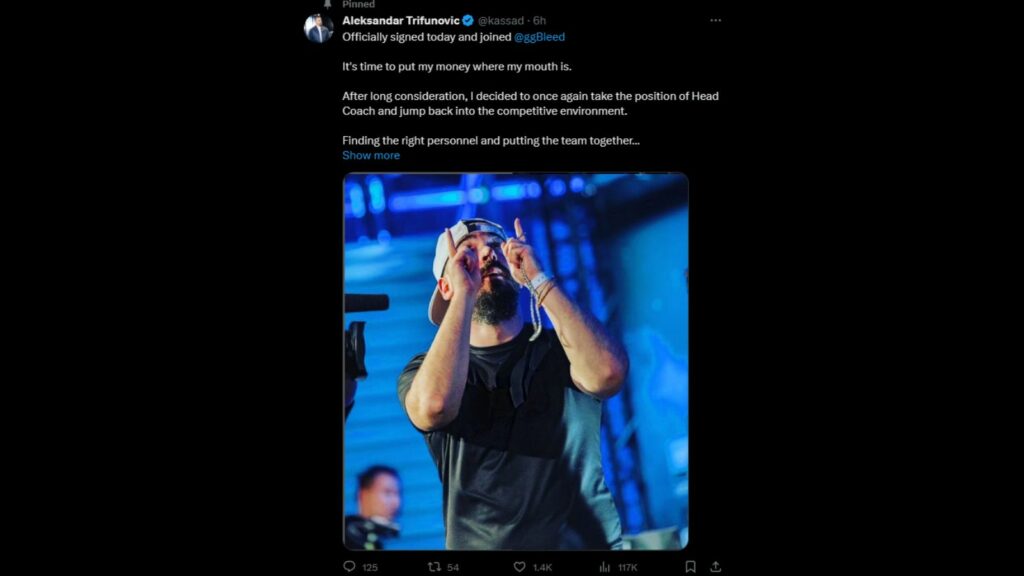**Description:**

This image depicts a tweet in a dark mode setting, characterized by a black background framing the content. The tweet itself is centered, flanked by substantial vertical black borders on the left and right. At the top left corner of the tweet, the word "Pinned" is highlighted, indicating it has been prioritized on the profile.

The tweet originates from a user named Aleksandar Trifunovic, spelled A-L-E-K-S-A-N-D-A-R T-R-I-F-U-N-O-V-I-C. His profile picture presents a man clad in a blue jacket. His Twitter handle is @Kasad (K-A-S-S-A-D). 

The tweet reads: "Officially signed today and joined GG Bleed. It's time to put my money where my mouth is. After long consideration, I've decided to once again take the position of head coach and jump back into the competitive environment, finding the right personnel and putting the team together."

Below the text, there's an option to "Show more," accompanied by an image of a man wearing a black shirt and a white backwards cap. The individual is gesturing with two fingers pointed upwards, his arms raised in front of him, adding a visual flair to the announcement.